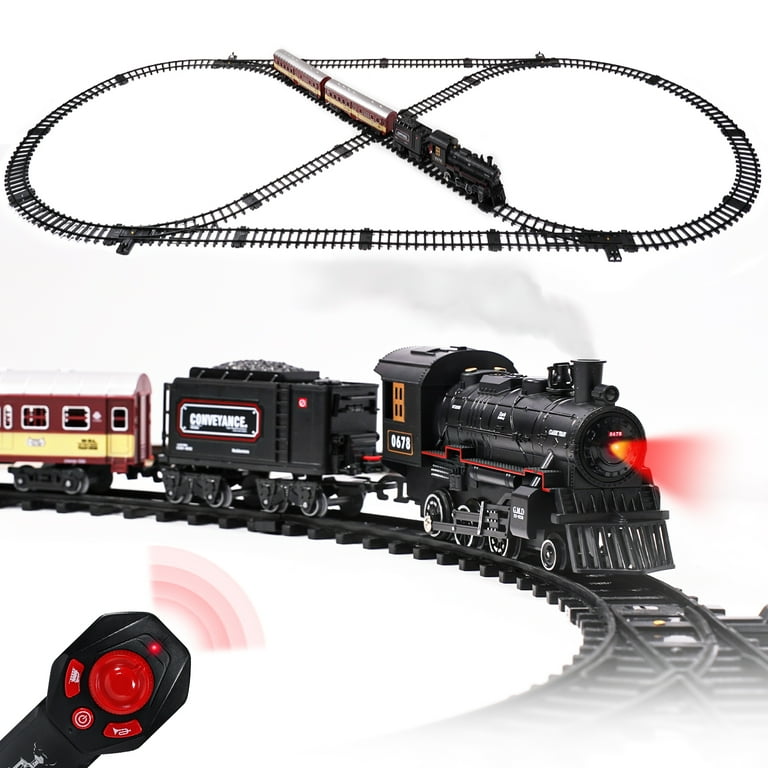The photograph displays a model railroad train set in two sections. The top portion of the image showcases the full layout of the tracks set up in an oval configuration with a figure-eight incorporated inside. The train is seen traveling from the top left to the bottom right on the figure-eight section. The close-up below provides a detailed view of the train engine, revealing its functional red headlamp at the front and the number 0678 marked on its rear. The engine is black, followed by a black car inscribed with the word "conveyance," likely for carrying coal, and a dual-colored passenger car with a silver top, light yellow body, and maroon red accents. The detailed front shot of the engine highlights its protruding red light and intricate design elements like the valves and grid iron. Surrounding the train is a white background, with a black and red remote control visible in the lower left, suggesting the ability to control the train’s lights, horn, and speed wirelessly.